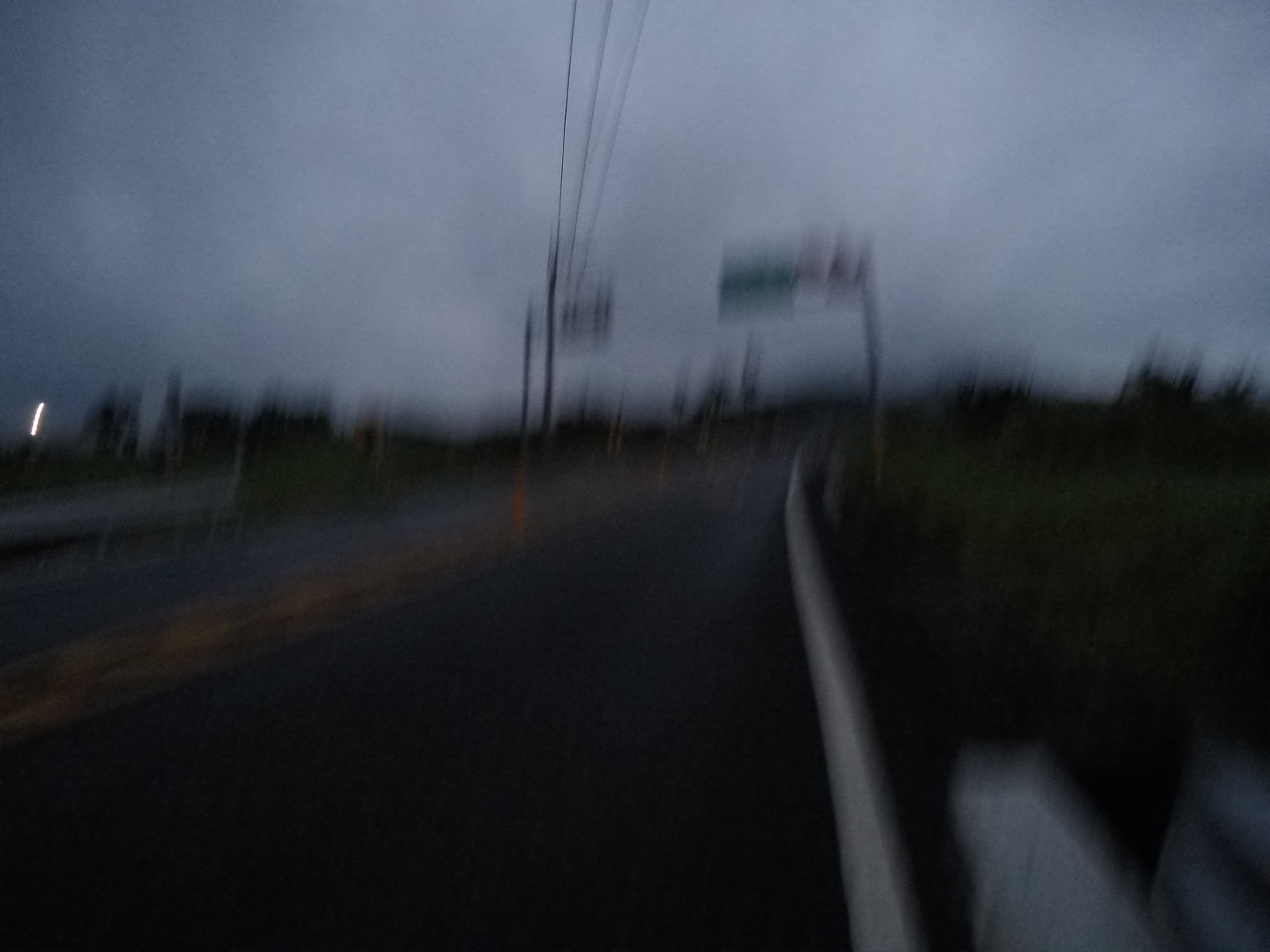The photograph, taken outdoors on a road, is notably blurry and was shot in a dimly lit location, obscuring many fine details. Despite the lack of clarity, a light silver or gray line meanders through the image, likely a metal guardrail lining the roadside. Prominently featured is a large metal pole, from which a green rectangular road sign hangs. In the background, hazy silhouettes of trees can be discerned, softened by the image's blurriness. A single light source illuminates the background faintly. Overhead, high electrical or telephone wires run parallel to the road, adding to the sparse infrastructure captured in the photograph.